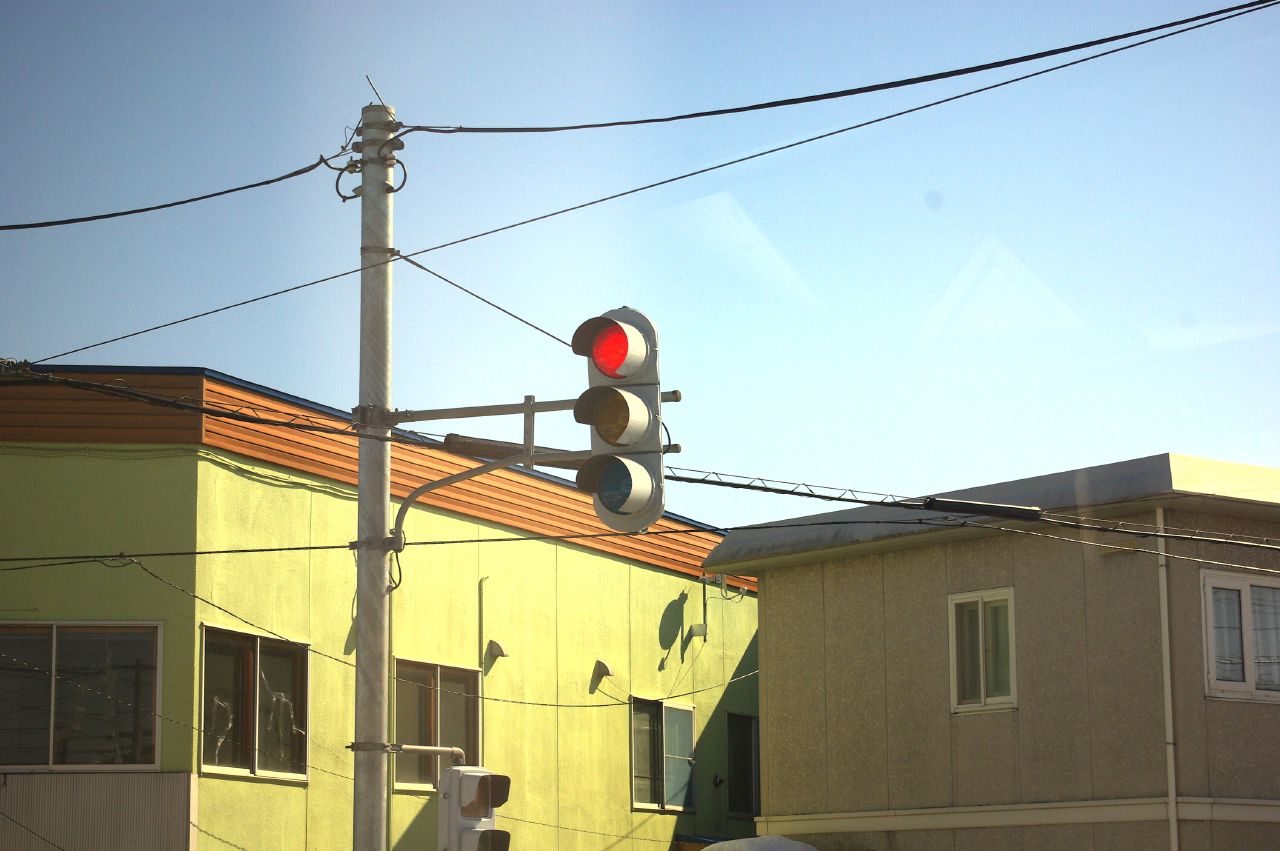This color photograph captures a traffic signal with a distinctive, rounded, pillow-shaped housing made of gray metal, currently displaying a glowing red light at the top. The traffic signal is mounted on a silver metal pole, from which numerous power lines extend, and a utility pole stands nearby. The backdrop reveals a clear blue daytime sky with a few white clouds. Two buildings are visible: one on the left is green with an orange border at the top and the other on the right is beige-brown with a silvery trim. Both buildings are square with flat roofs and appear to be two stories high. The green building has numerous windows, some of which are broken and taped over, while the beige-brown building features a small rectangular window on the front and a couple on the sides. There are no people, animals, or motorized vehicles visible in the photograph.